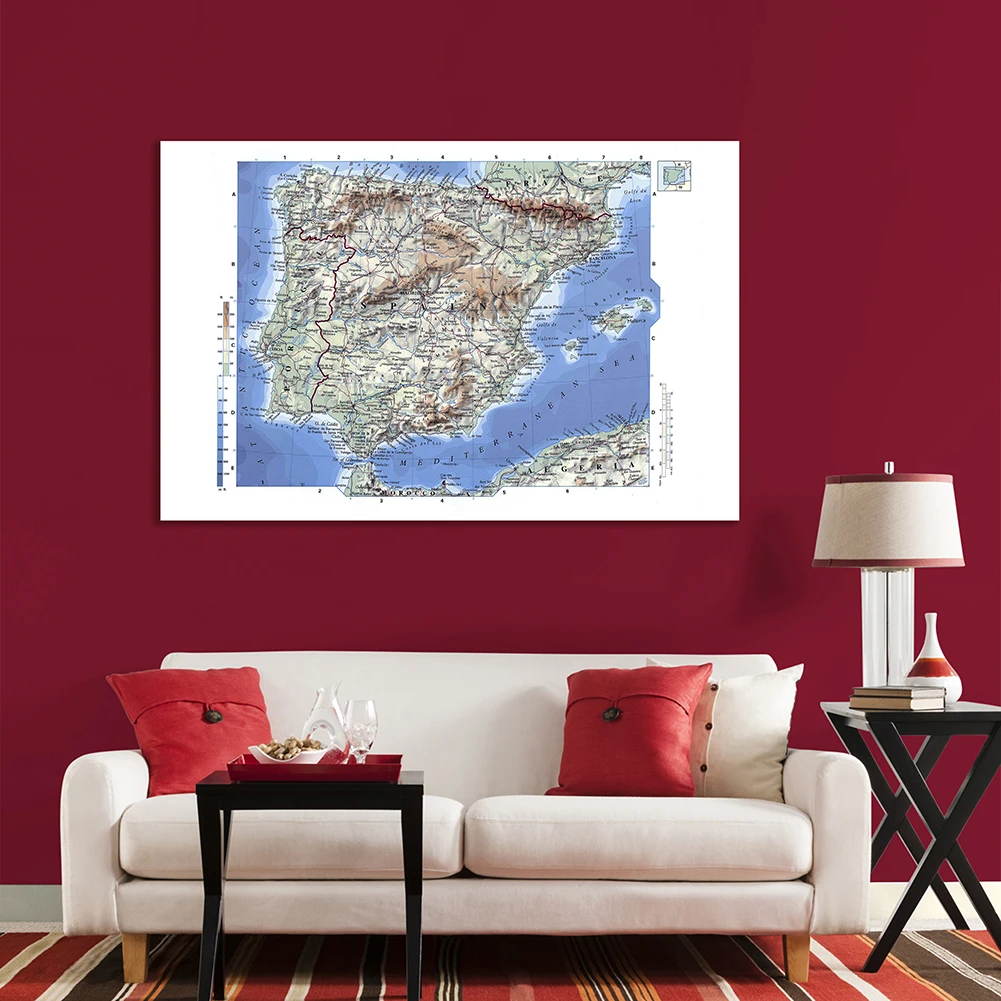In this indoor living room scene, the back wall is a vibrant maroon or burgundy red adorned with a horizontally-hung rectangular map. The map vividly shows the Mediterranean Sea, Atlantic Ocean, and various landmasses including Algeria and Spain, with discernible topography of deserts and mountains. Below the map, a white leather couch is positioned, accented with two large red pillows featuring brown buttons. In front of the couch, there's a small coffee table that holds a red serving tray with a cup and food, alongside two books. To the right of the couch stands a fold-out table with a vase, a cup, and a unique lamp. The lamp has a white base and a shade that is predominantly white with red burgundy strips on the top and bottom. The floor is covered with an orange, white, and brown striped carpet that is not uniformly patterned. The bottom trim of the wall is white, completing the room's cohesive yet detailed decor.